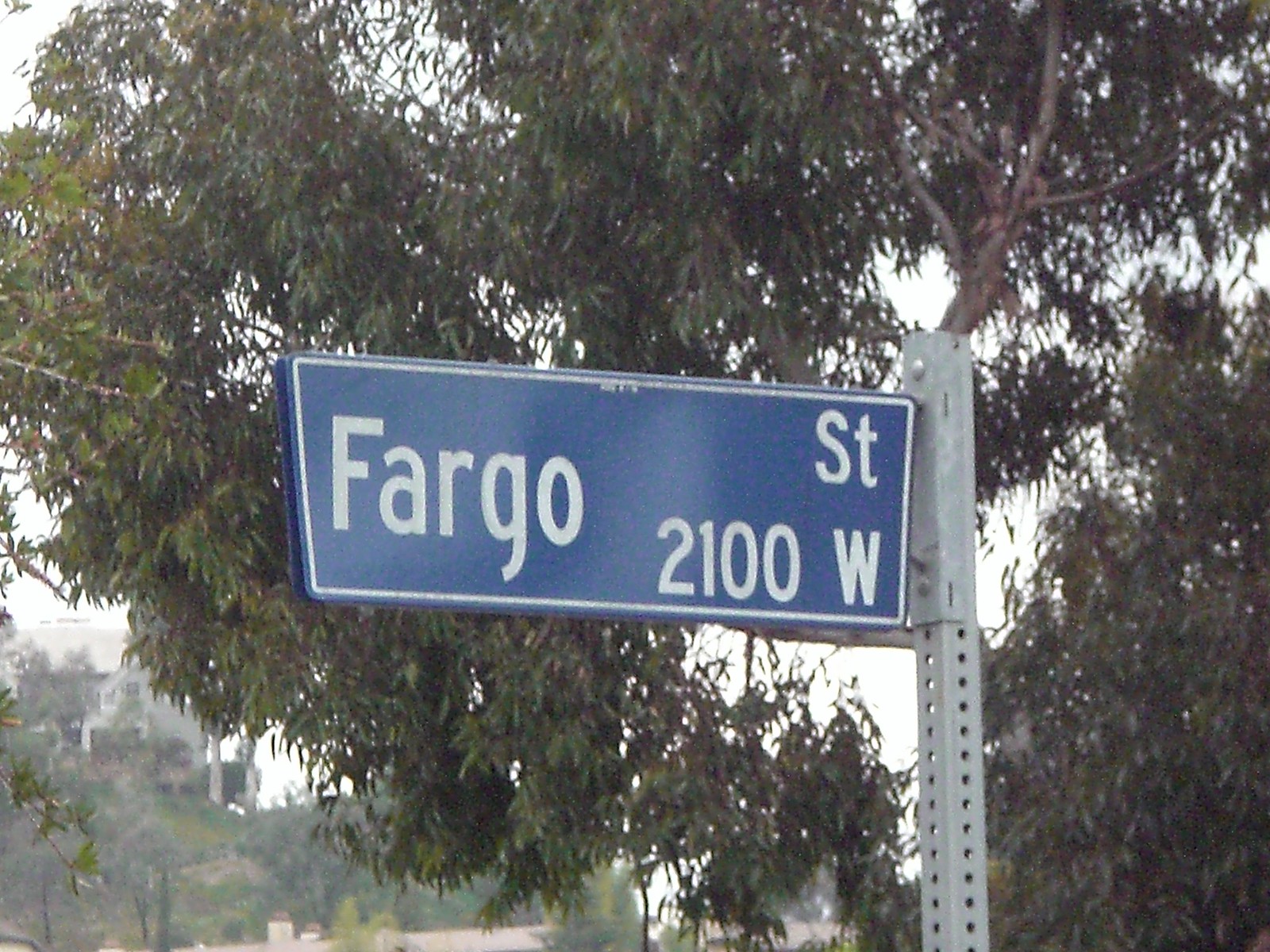In the image, there is a street sign mounted on a square metal pole with adjustable-height perforations. The sign displays "Fargo 21" and "Fargo Street 2100 West." Just behind this sign, there appears to be a second, identical sign facing the opposite direction, creating a doubled effect. A verdant tree with green leaves stands prominently in the background. Beyond the tree, there's a white building surrounded by sandy ground, additional vegetation, and more trees.